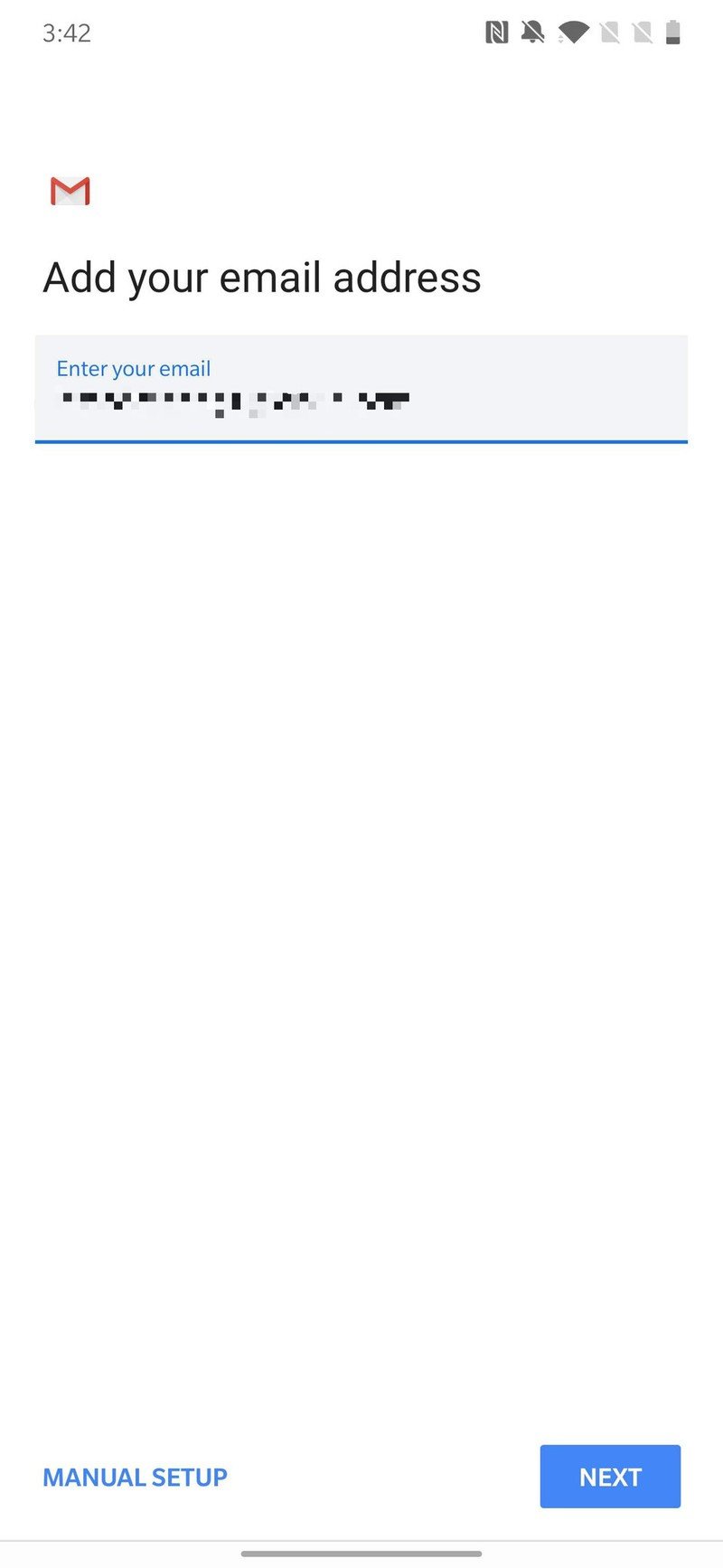Screenshot of a mobile device screen, depicting the process of adding a Google email account. At the top, the status bar displays critical device information. The battery level is critically low, and no SIM cards are installed, as indicated by two crossed-out SIM card icons. The device has a full Wi-Fi signal, and the volume is muted, shown by a struck-through bell icon. The current time is 3:42.

The main focus of the screenshot is the Google account setup interface set against a white background. In the upper left corner is the red Gmail logo, followed by the instruction "Add your email address" in black text. Below this, there's a light blue input box with the text "Enter your email" in blue, within which an email address has been entered but is blurred out for privacy. Two buttons are present at the bottom: "Manual setup" in plain text on the left, and a blue "Next" button with white text on the right.